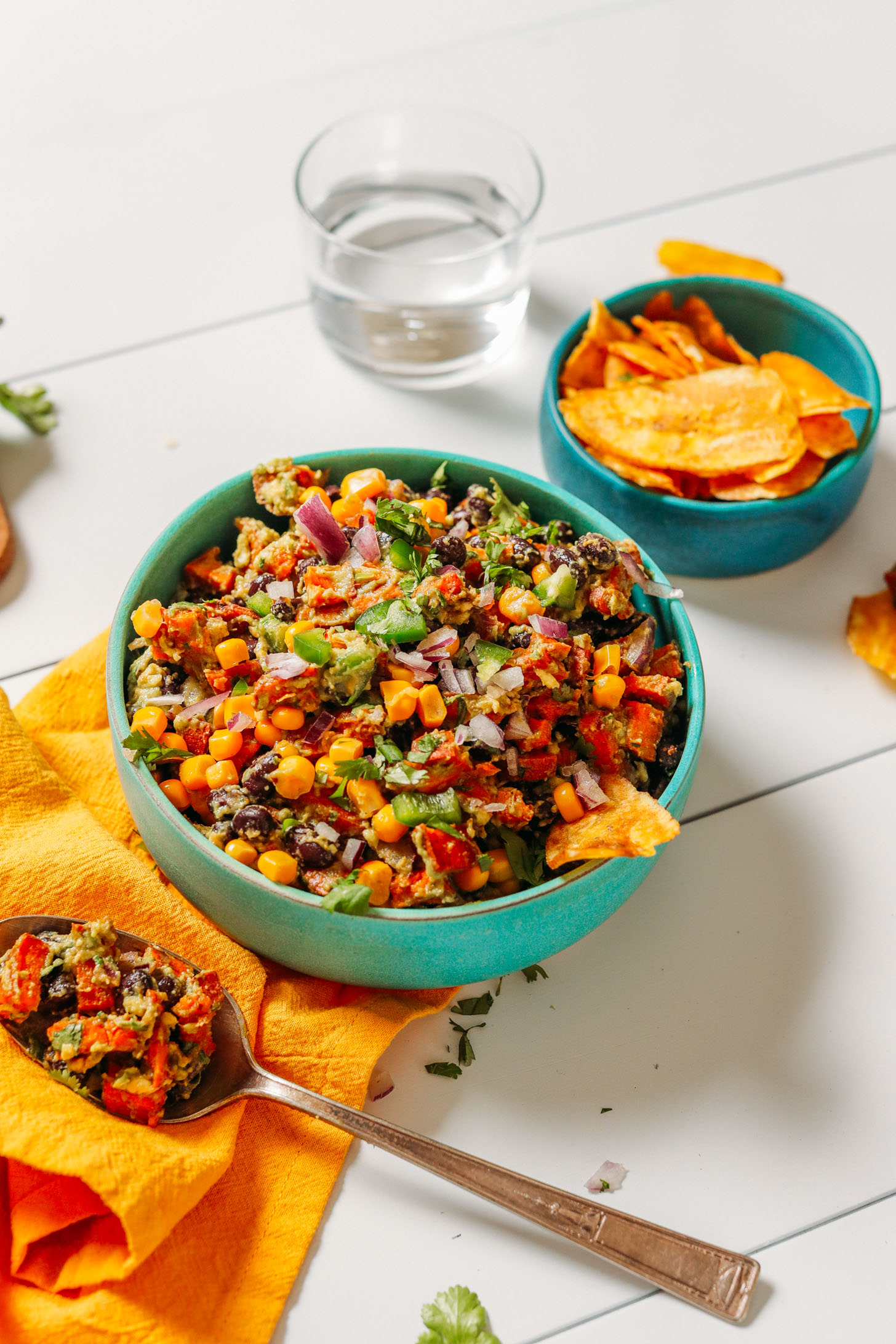The vertically aligned rectangular image depicts a vibrant picnic table, painted white, with visible wood slats. At the center of the table, a striking green bowl with a gold rim holds a colorful dish. This dish appears to be a zesty mixture, likely a dip or salad, featuring ingredients such as black beans, corn, diced tomatoes, red and green onions, bell peppers, and possibly celery and parsley. To the upper right of this bowl, a teal blue bowl contains large, triangular orange tortilla chips. Positioned at the top middle, a small, transparent glass is half-filled with a clear liquid, possibly water. On the bottom left corner of the table, an orange dish towel rests with a silver-handled spoon on it, holding a spoonful of the vibrant mixture from the green bowl.